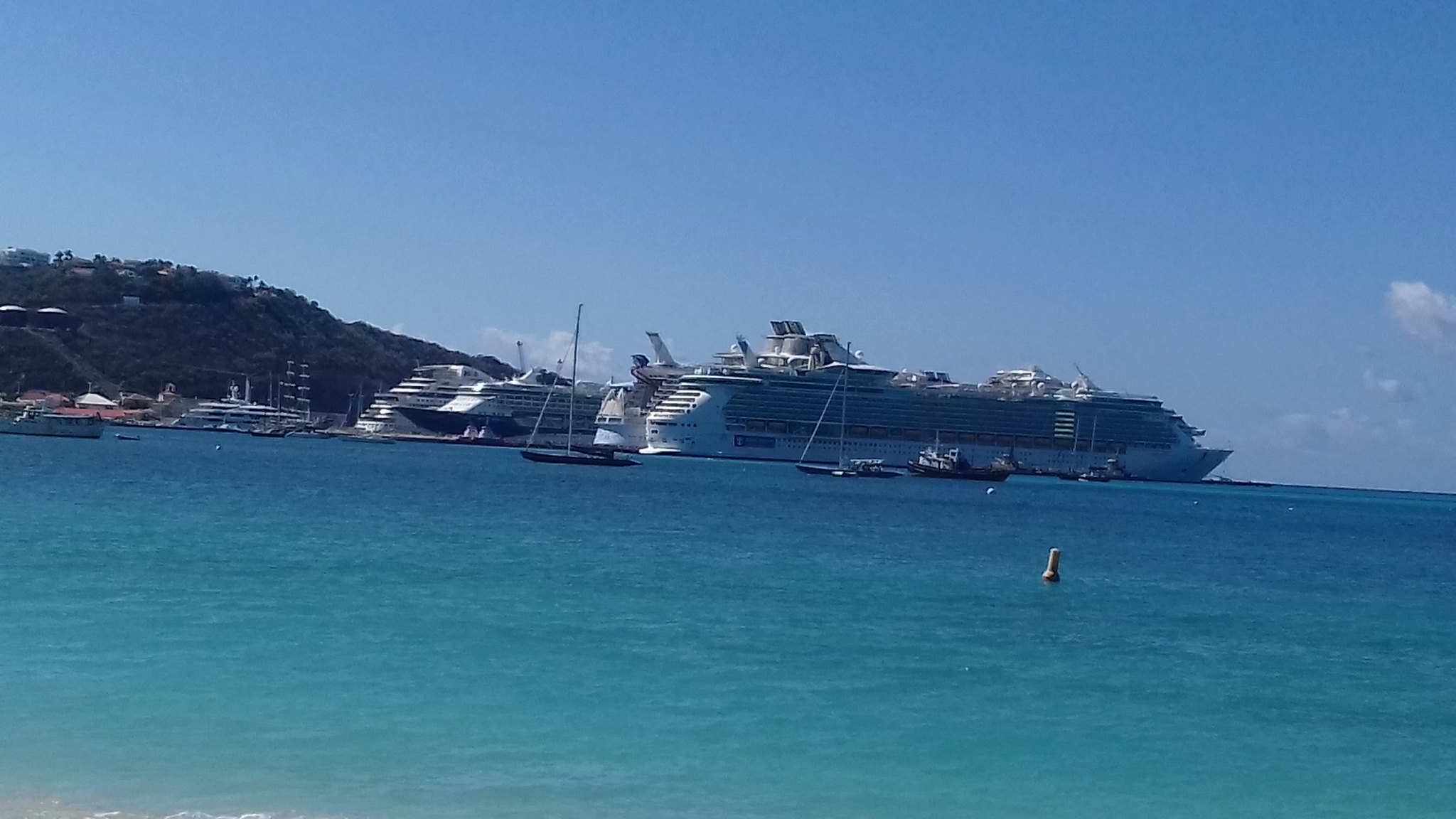This photograph captures a tropical bay from a coastal viewpoint, showcasing four large, white cruise ships docked side by side offshore against a backdrop of turquoise water and a deepening blue sky. Each cruise ship boasts multiple floors, potentially as many as ten, with numerous windows and bustling activity on their decks. In the foreground, the sea transitions from a white sandy shore to a deeper teal hue, marked by a buoy midway to the horizon. Smaller vessels, including yachts, sailboats, and a black boat, dot the water between the cruise ships and the beach. To the right, a dark, tree-covered hillside slopes down towards the water, with tiny specks hinting at distant houses. White clouds drift just above the horizon, enhancing the scenic, tropical ambiance of this detailed, nautical vista.